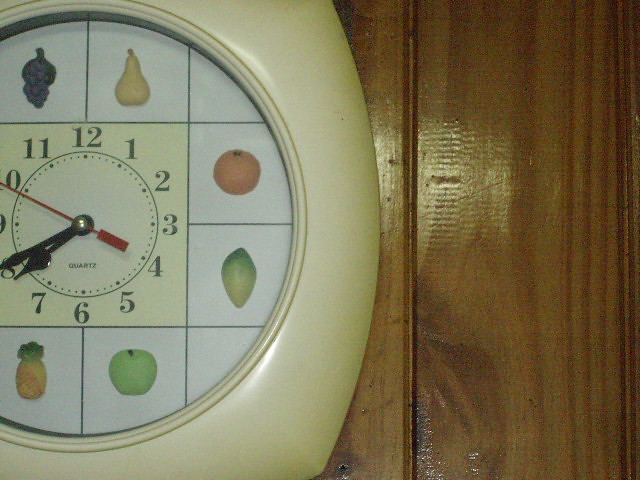This photo features a retro kitchen wall clock with a design reminiscent of the 1970s or early 1980s. The clock is encased in an ivory-colored plastic frame with an oval vertical shape and squared edges. Set within this frame, a square inset houses the round clock face, which prominently displays the word "quartz." The clock's face is adorned with black Arabic numerals and black hour and minute hands that point to 7:40. A distinctive red second hand is positioned at the 50-second mark. Behind the clock face is a decorative grid featuring illustrations of various fruits: grapes and a pear at the top, an orange in the next row, an avocado in the following row, and a pineapple and an apple at the bottom. The clock is situated on the left side of the image. To the right, there is paneling that appears to be from an older building, several decades old, with a sheen that suggests a light source in the foreground, giving it a shiny, shellacked appearance.